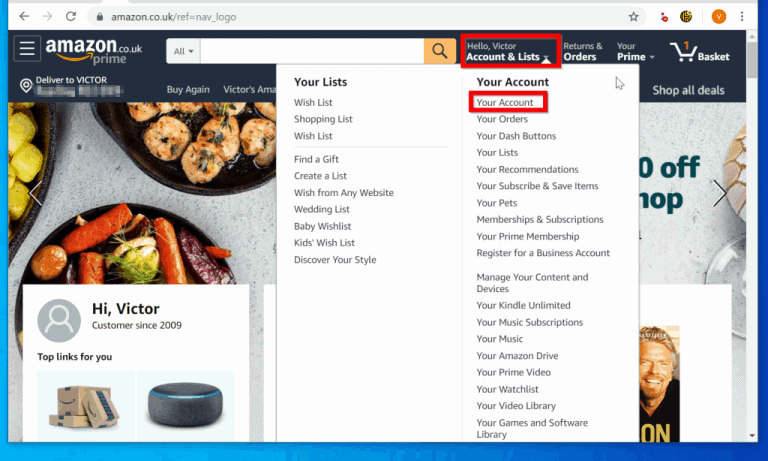The image depicts the Amazon website, either amazon.com or amazon.co.uk, prominently featuring a blue banner in the top-left corner that reads "Amazon Prime." To the left of this banner is a hamburger menu icon labeled "Deliver to Victor," though additional information is not displayed. The top navigation bar includes the greeting "Hello Victor," followed by the "Accounts and Lists" drop-down menu.

When the "Accounts and Lists" menu is expanded, several options are visible: "Your Lists" encompasses categories like Wish Lists, Shopping Lists, Find a Gift, Create a List, Wish for Many Websites, Wedding Lists, Baby Wish Lists, Kids Wish Lists, and Discover Your Style. The account section further includes links to "Your Orders," "Your Dash Buttons," "Your Recommendations," "Your Subscribe and Save Items," "Your Pets," "Memberships and Subscriptions," "Your Prime Membership," "Register for a Business Account," "Find Your Content and Devices," "Your Kindle Unlimited," "Your Music Subscriptions," "Your Music," "Your Amazon Drive," "Prime Video," "Your Watchlist," "Your Video Library," and "Your Games and Software."

The image highlights Victor’s long-standing relationship with Amazon, as he has been a customer since 2009, and showcases the tailored links and options available to him, reflecting his frequent use of the platform. The sentiment "Amazon loves Victor" summarizes the personalized experience displayed.